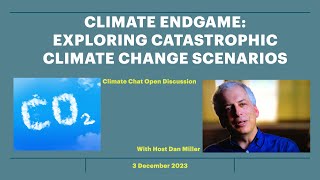The image is a rectangular banner advertising an event, with the top and bottom sides twice as long as the left and right sides. The background is a dark blue. At the top, in white text, it reads "Climate Endgame: Exploring Catastrophic Climate Change Scenarios." Centered beneath this, smaller yellow text announces "Climate Chat: Open Discussion with Host Dan Miller, 3 December 2023." To the left, there is a small picture of clouds on a blue sky with the text "CO2." On the right, there is a photograph of an older man with white hair, wearing a blue button-up shirt, visible from his shoulders upwards. He appears to be talking, and behind him is a window and a brown and tan colored wall.